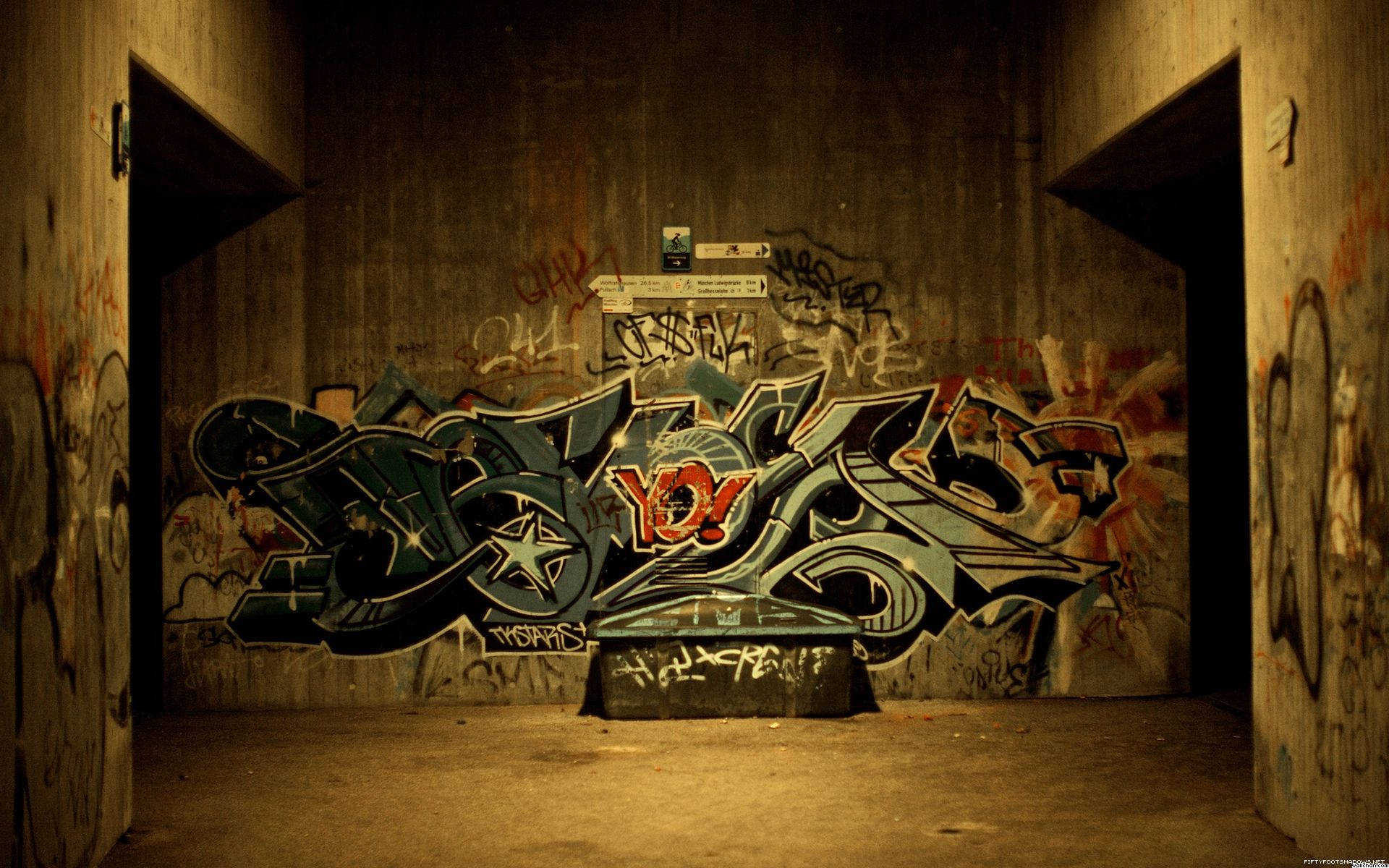The photograph appears to be taken at night in an industrial or possibly abandoned underground area, characterized by concrete walls that extend into dark passages. The space has the feel of somewhere rarely traversed, such as beneath a bridge or even within a sewer system. The most striking feature of the image is the extensive graffiti art covering the concrete walls. Dominant among the various tags and scribbles is an elaborate piece rendered in light blue and black bubble letters, adorned with a star and a cloud in the lower left corner. Despite the intricacy, much of this graffiti is difficult to decipher. Notably, the word "YO!" is prominently painted in red, with an exclamation point adding emphasis. Additional red initials, "GHK", are spray-painted nearby. The large, central graffiti piece is surrounded by smaller tags, indicating a possibly respectful acknowledgment of the main artwork. The myriad of graffiti styles and scribbled writings suggests contributions from different individuals, lending a sense of layered urban artistry to the scene.